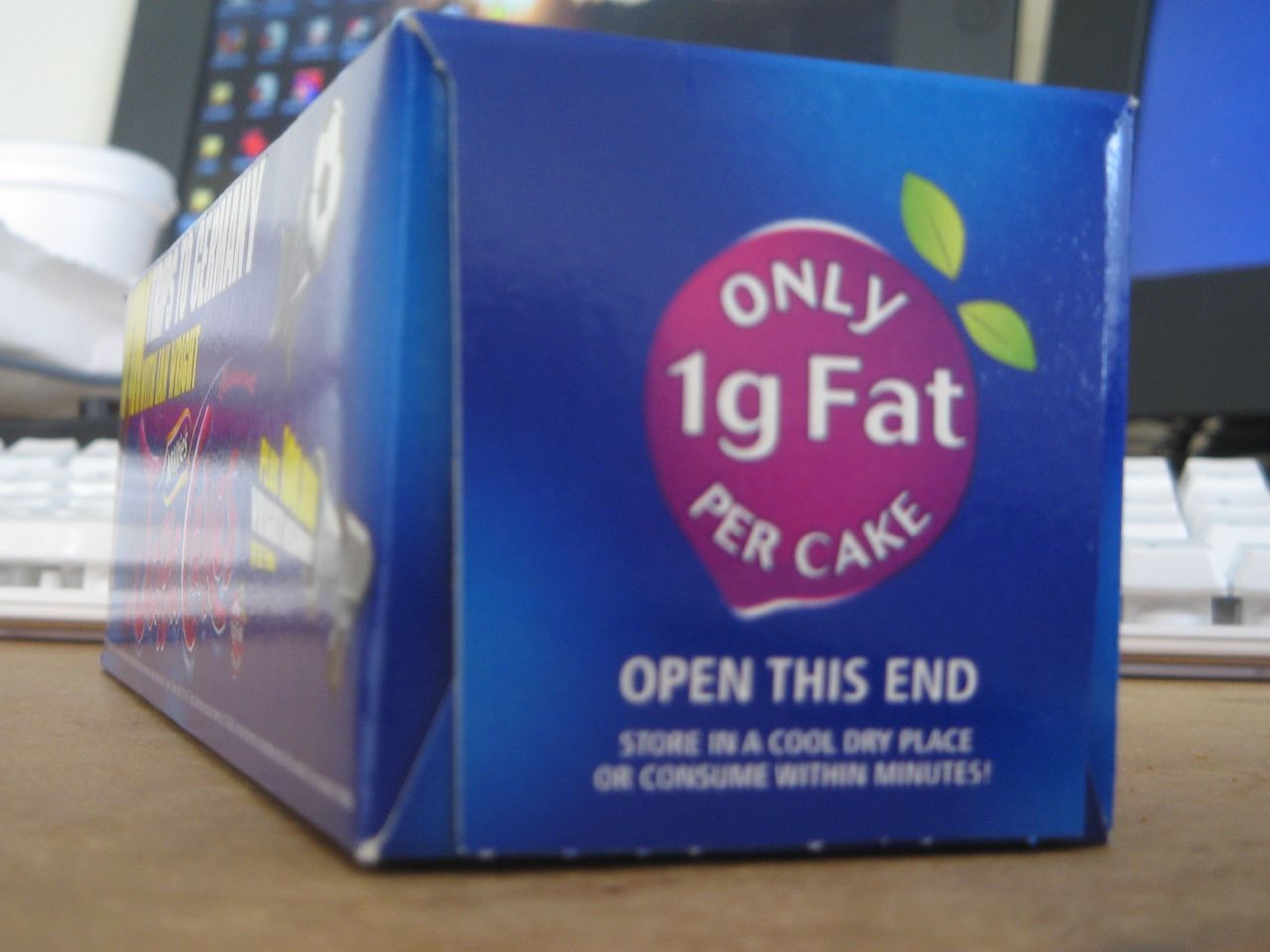The image captures a dark blue rectangular box positioned on a surface, possibly a carpet or table. The side of the box facing the viewer displays a red circle with white text inside that reads, "Only 1g fat per cake." This circle is accented with two small green leaves, adding a subtle touch of nature or healthiness to the design. Adjacent to this red circle, the box instructs, "Open this end, store in a cool, dry place or consume within minutes." 

Towards the front of the box, which is partially out of view and facing left, there appears to be text hinting at a possible German origin, although the exact wording is unclear. The box's front is adorned with yellow and white lettering and features a red, squiggly element, contributing to a vibrant and enticing visual presentation.

In the background, a white keyboard and a computer monitor with visible icons suggest that the box is located on a computer desk, implying that it contains snacks or other consumables suitable for a work or home office setting. The overall scene combines elements of daily life with the promise of a light, low-fat treat.